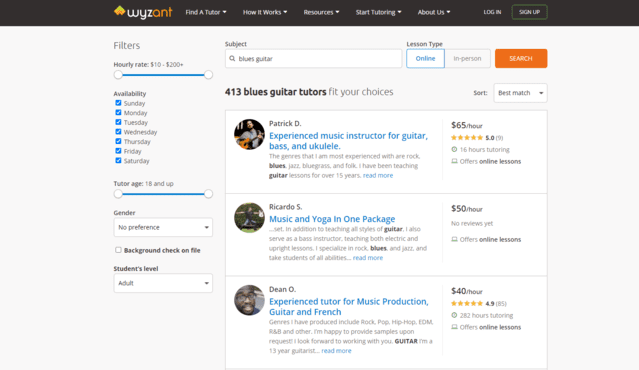This image displays the homepage of the "WyZant" website, featuring their name prominently at the top. The word "WyZ" is in a distinct white font, while "ant" is styled in a reddish-orange color, all set against a black navigation bar. To the right of the "WyZant" logo, there are several tabs: "Find a Tutor," "How it Works," "Resources," "Start Tutoring," "About Us," "Log In," and "Sign Up." Further to the right, there's a downward-facing arrow indicating a drop-down menu.

The main background of the page is white, with a filter section on the left side, which includes various sliders, checkboxes, and additional drop-down menus for refining search results. In the central section, it is noted that there are "413 blues guitar tutors" that match the chosen filters. On the right side, there is a sorting box available for further organizing the displayed results.